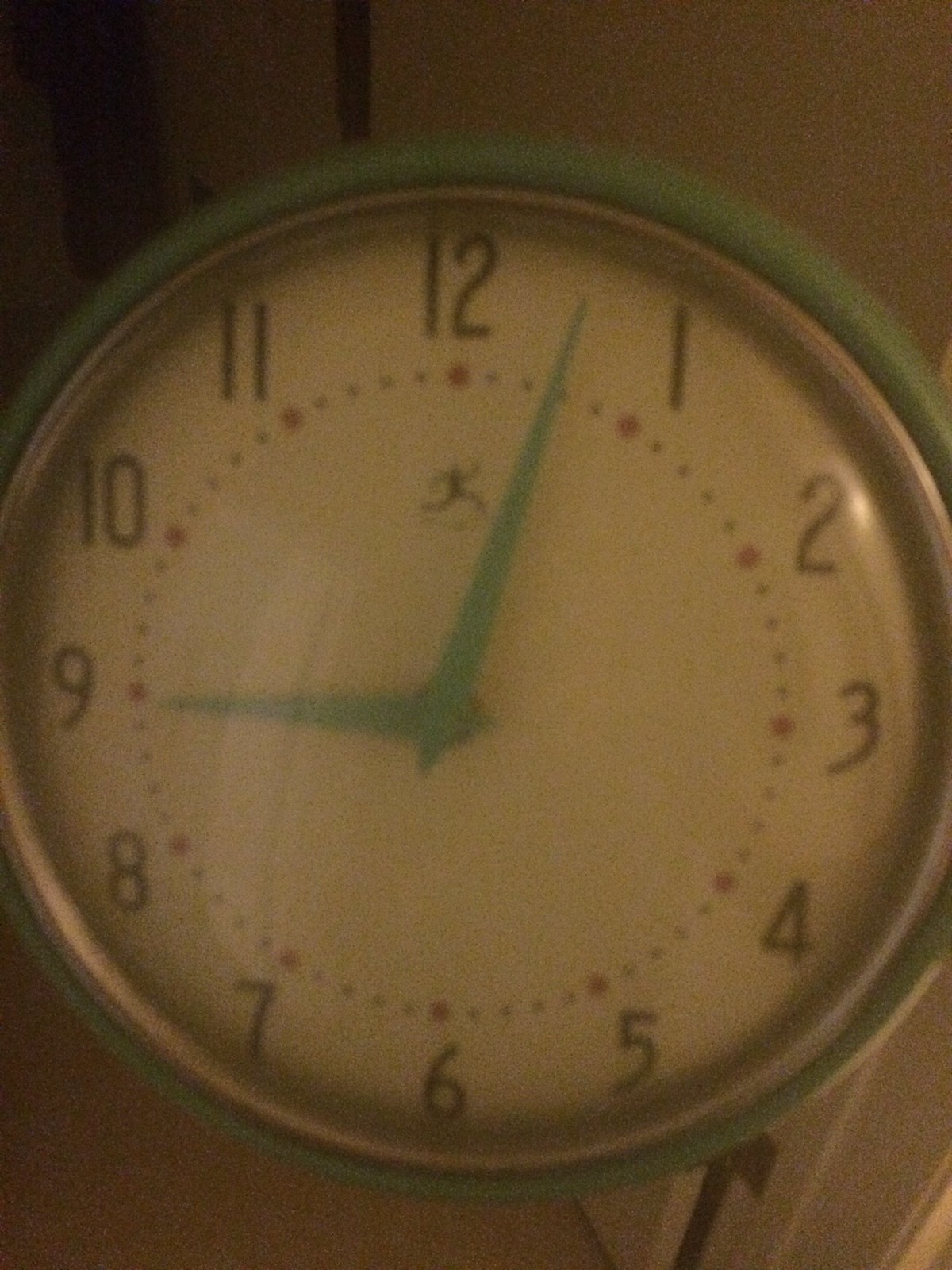This is a close-up image of a wall clock. The clock features a thick green border encompassing its circumference, adding a vibrant touch to its overall design. Protecting the clock face is a silver-rimmed glass cover, enhancing its sleek appearance. The clock's hands are green, indicating the time as approximately 9:03. Large, black numerals mark each hour, aiding in easy readability. Surrounding the clock's center are decorative dots: larger red dots positioned at each hour mark and smaller black dots indicating the minutes. Above the numeral 12, there is an illustration of a running man, adding a unique character to the clock. In the background, toward the bottom right, a door hinge and a portion of a doorway frame are visible. On the bottom left, part of the ground can be seen, though it is very dark and lacks distinguishable details. Overall, the dim lighting casts a shadow over much of the image, contributing to its mysterious ambiance.